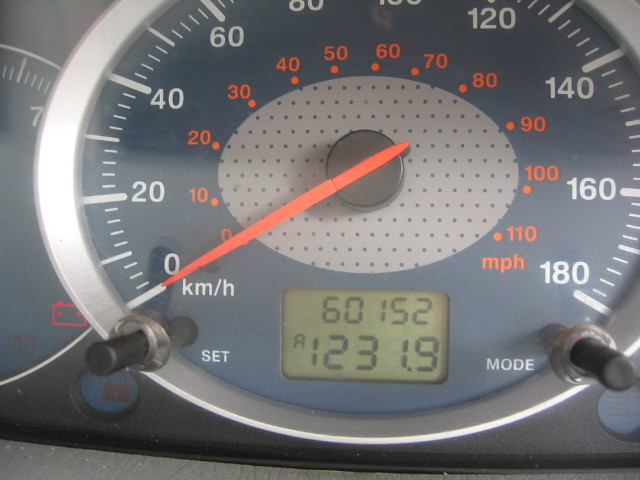This image captures the detailed interior of a vehicle, focusing specifically on the speedometer. The speedometer is prominently oval-shaped with a sleek silver outline. Its face is a deep navy blue with crisp, white numbers arranged in a circular fashion, starting from 0 and going up to 180, indicating kilometers per hour (KM/H) as labeled at the zero mark.

Nested within the main speedometer is a smaller, oval-shaped gauge featuring a gray background with blue dots. This inner gauge uses an orange font to display numbers from 0 to 110, explicitly marked for miles per hour (MPH) below the 110 indication.

An orange-colored needle points out the current speed in both kilometers and miles per hour. Below the needle, a digital display details the car's mileage, currently showing 60,152 miles. Another figure, 1,231.9, likely represents the distance tracked for a specific trip or journey. The entire setup is both functional and aesthetically coordinated, providing clear readability for the driver.